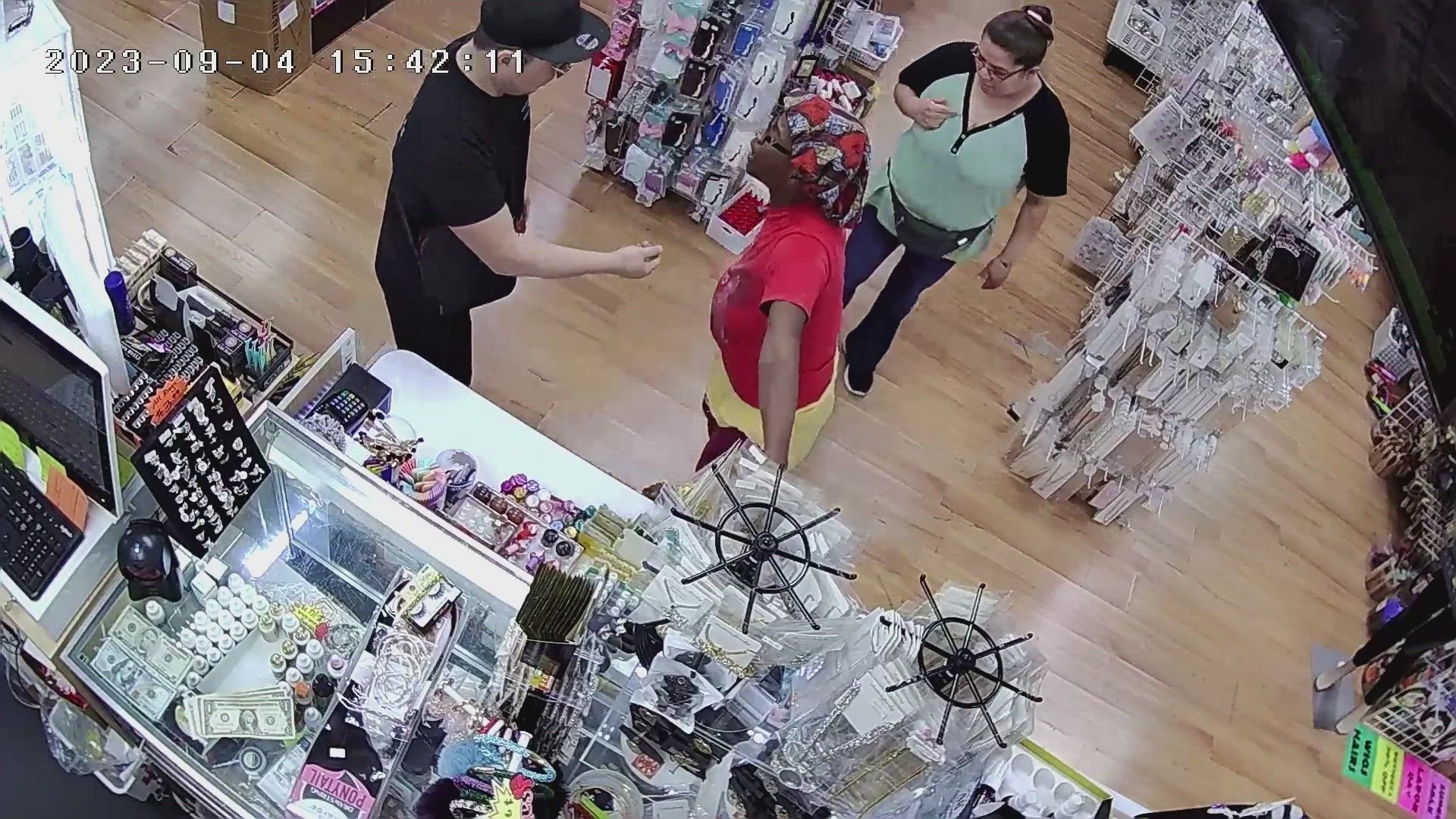The high-resolution colored security camera footage, dated September 4th, 2023 at 3:42:11 PM, captures a heated argument inside a retail store, likely an accessory or beauty supply store, given the items visible on racks and the cashier's counter. The timestamp is prominently displayed at the top left corner of the image. The store features a glass countertop, a computer display, a keyboard, and money on the counter. 

In the foreground, a man dressed in all black, including a hat, t-shirt, pants, and an over-the-shoulder bag, extends his right hand as if expecting something from the woman opposite him. The woman, appearing aggressive and argumentative, wears a floral cap, glasses, a red shirt, and a yellow skirt. 

Behind and slightly to the right of this woman, another bystander stands observing the confrontation. She has her hair pulled back, wears glasses, a black and light green shirt, a black fanny pack, denim pants, and black sneakers. The store layout, with accessories and beauty supplies around the cashier area, suggests a setting designed for small, personal items, accentuated by the wooden flooring.